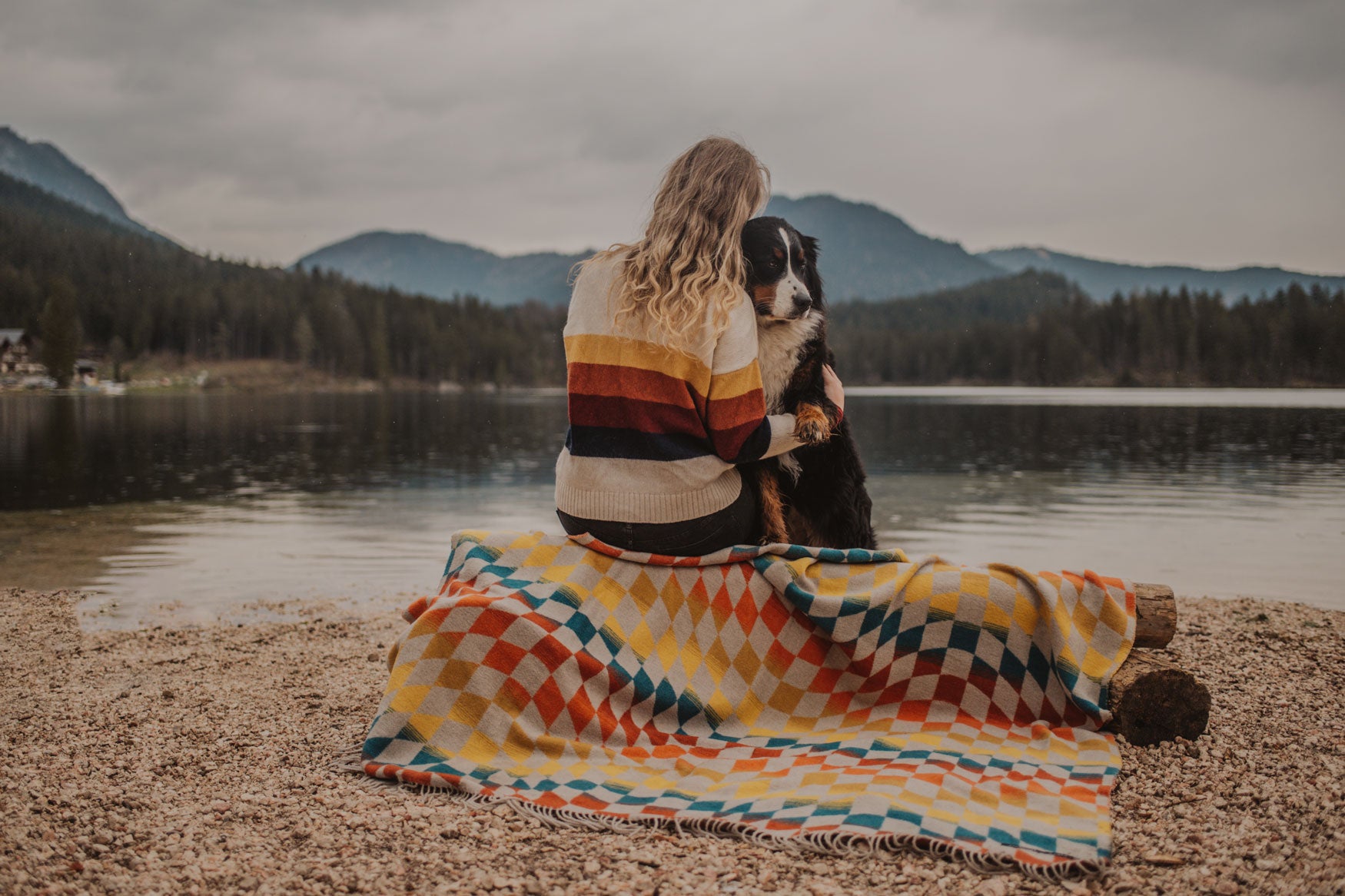A serene lakeside scene captures a woman with curly blonde hair and her shaggy, tricolored dog, likely an Australian shepherd, cozied up on a log. They are wrapped in a vibrant blanket with a checkerboard pattern in shades of gray and a rainbow gradient, complementing the woman’s colorful sweater with horizontal stripes of yellow, orange, red, brown, and blue. The woman, seen from behind, embraces her dog, who rests his head on her shoulder. The tranquil setting includes calm lake waters framed by dense pine trees and majestic mountains under an overcast, gray sky, hinting at a chilly autumn day, perfect for snuggling.